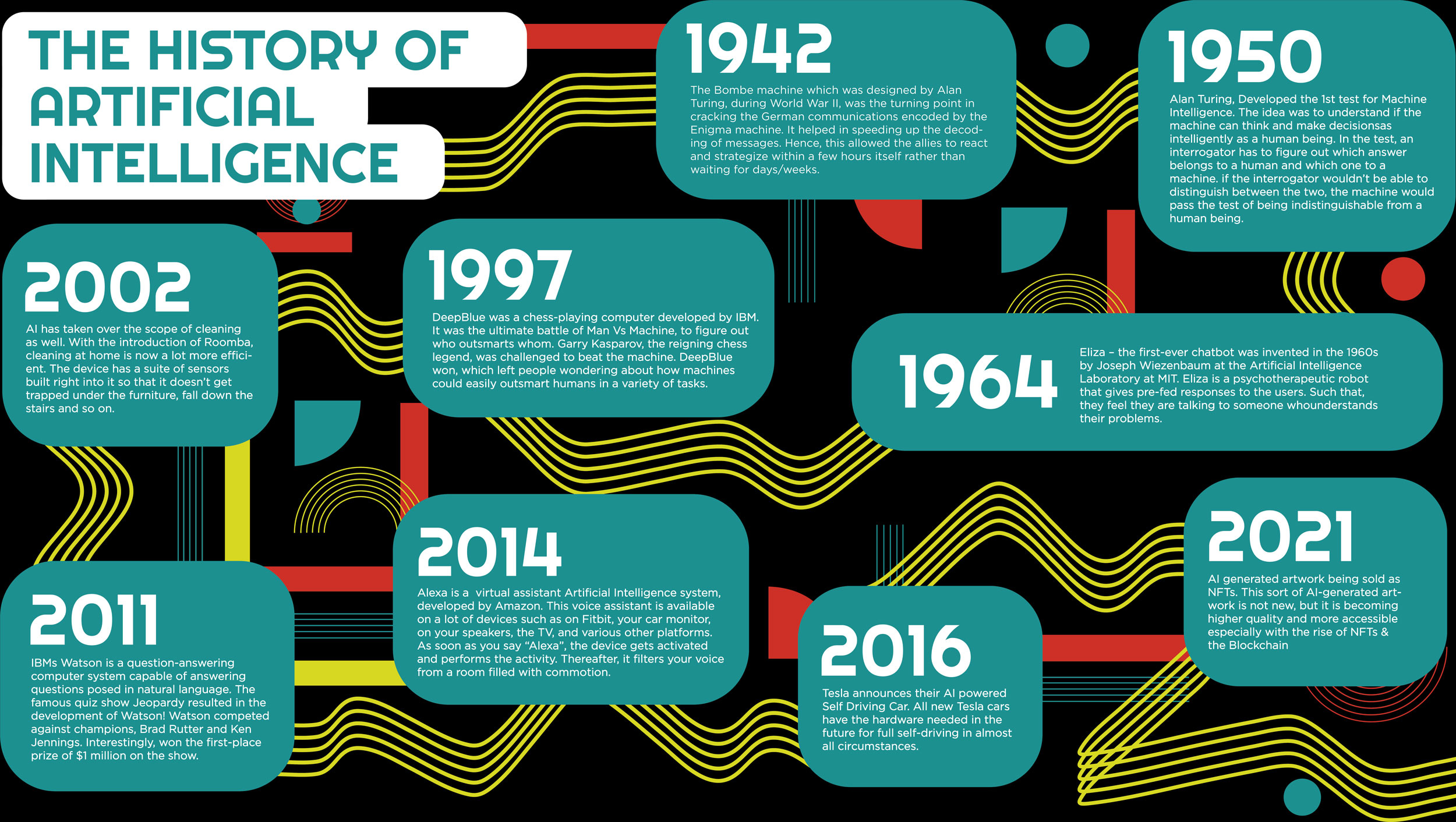The poster titled "The History of Artificial Intelligence" features a black background with curving yellow lines connecting various teal and red boxes, each highlighting significant milestones in AI history. This timeline begins in the center with the year 1942 and continues chronologically to 1950 and 1964, moving to the right before looping back to the left. Key years such as 1997, 2002, 2011, 2014, 2016, and 2021 are marked, each accompanied by paragraphs of white text that detail important developments within those years. The intricate design, which resembles a textbook spread, serves to map out the evolution of artificial intelligence from its early stages to recent advancements, with yellow lines and various color-coded boxes guiding the viewer across the poster's rich summary of AI's transformative journey.